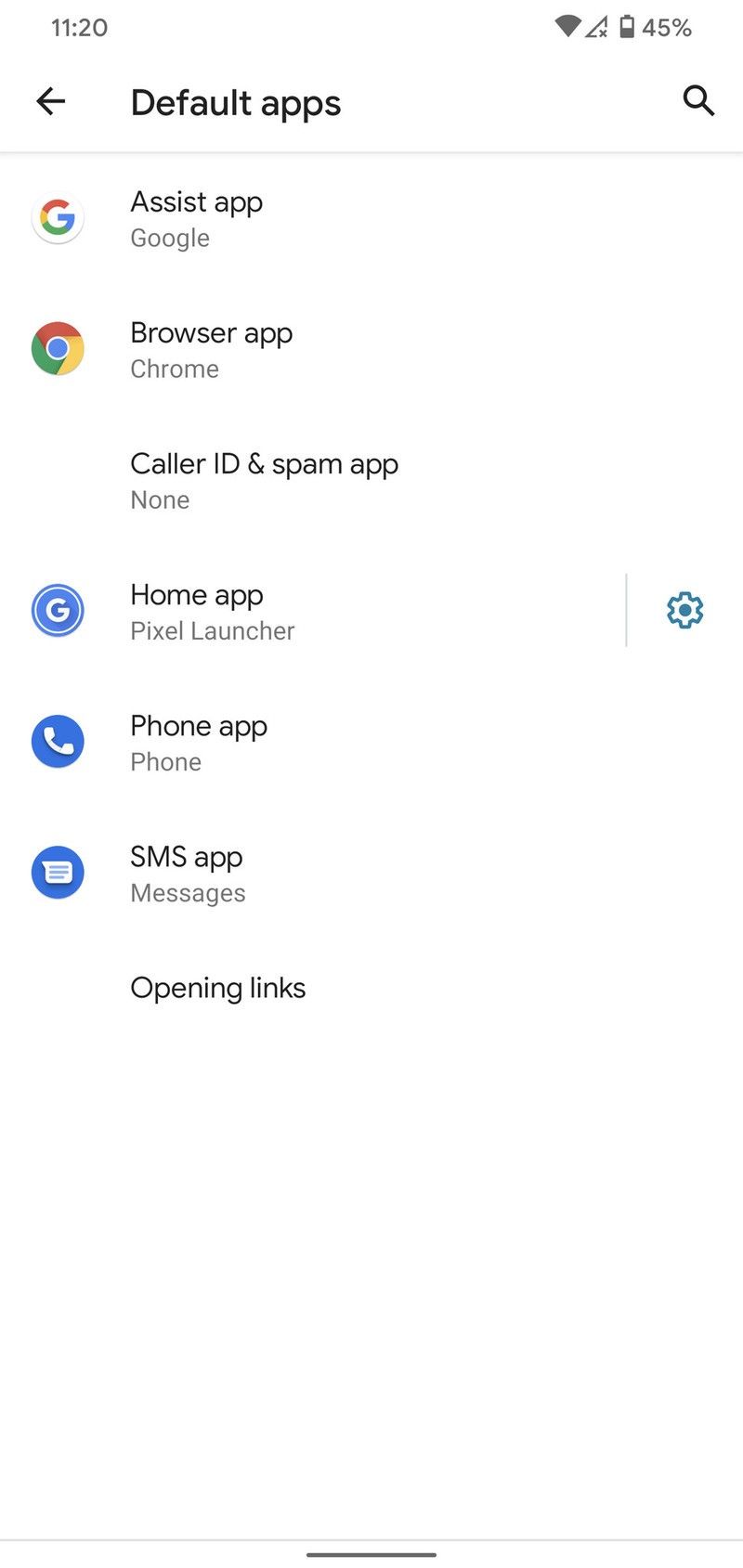This screenshot depicts an application interface on a smartphone, showcasing the default apps settings screen. At the top of the screen, there is a back arrow icon, a magnifying glass icon for search functionality, and the title "Default Apps." The smartphone’s status bar at the very top displays the time as 11:20 AM on the left side, and on the right side, indicators include full signal strength, a triangular icon, and a battery level icon showing 45% charge.

Beneath the header, the screen lists various default applications each accompanied by their respective icons on the left and their names on the right. The listed apps include:
1. Google Assistant with its recognizable icon.
2. Chrome browser with its distinct multicolored circle icon.
3. Caller ID & Spam App, which appears to have its icon missing or set to "None."
4. Home App, represented by a blue 'G' icon.
5. Phone App, symbolized by a standard phone receiver icon.
6. SMS App, depicted with a text speech bubble icon.

The layout is presented on a clean white background with black text, maintaining a simple and user-friendly interface.